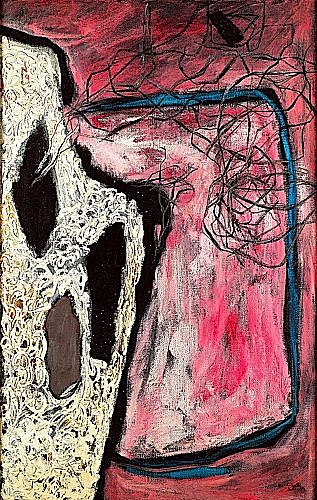The abstract painting, set against a black background, presents a striking display of random geometric shapes and bold colors. Dominating the left side, a white, rocky form features three small black holes. Adjacent to it, a black-outlined box extends, while the painting's central area is a blend of red hues mixed with streaks of white. The upper right portion is intricately adorned with jumbled black wire-like squiggles resembling tangled tubing, some of which seem to cascade into the black holes. In addition to the prominent reds, whites, and blacks, hints of brown, gray, pink, purple, and teal add to the visual complexity. The entire composition feels chaotic yet vividly expressive, embodying the quintessential essence of abstract art without any discernible objects or text.